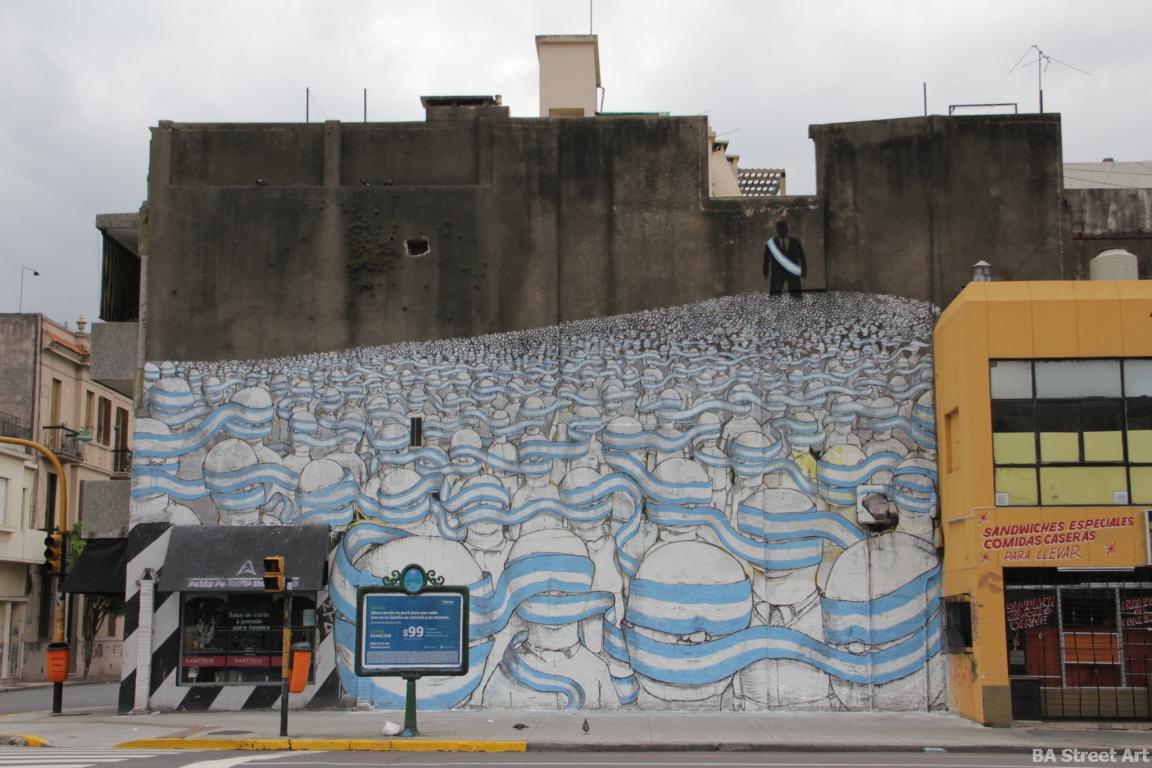This photograph captures an intricate mural on a gray concrete building situated at a street corner, complete with a sidewalk and a crosswalk in front of it and a large sign. The mural features an expansive display of numerous entirely white faces and figures, each dressed in white attire. Every figure in this congested crowd has their eyes and mouths obscured by a light blue and white banner. Dominating the top section of the mural is a striking image of a man standing, his face completely blacked out, and he dons a black suit with a sash made of the same blue and white banner. The mural is rich with blue hues interwoven with white, creating a powerful visual narrative centered on uniformity and concealment, emphasized by the repetitive use of the blue and white banner covering the faces of all the depicted characters.